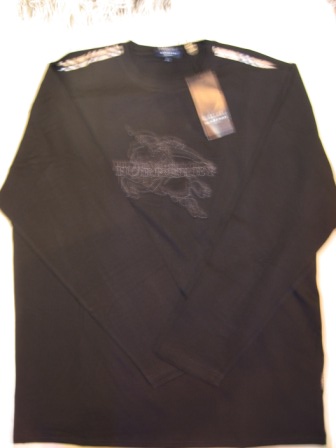A blurry image depicts a long-sleeve black shirt against a plain white background. The sleeves are crossed over the chest, subtly framing a white design on the front, which remains indistinct and appears to possibly feature an astronaut with some text, although the specifics are unclear. At the neckline, an orange and black product tag is visible, suggesting brand or sizing information. Additionally, white and orange stripes run from the neckline across the shoulders, adding a distinctive touch to the shirt's design.